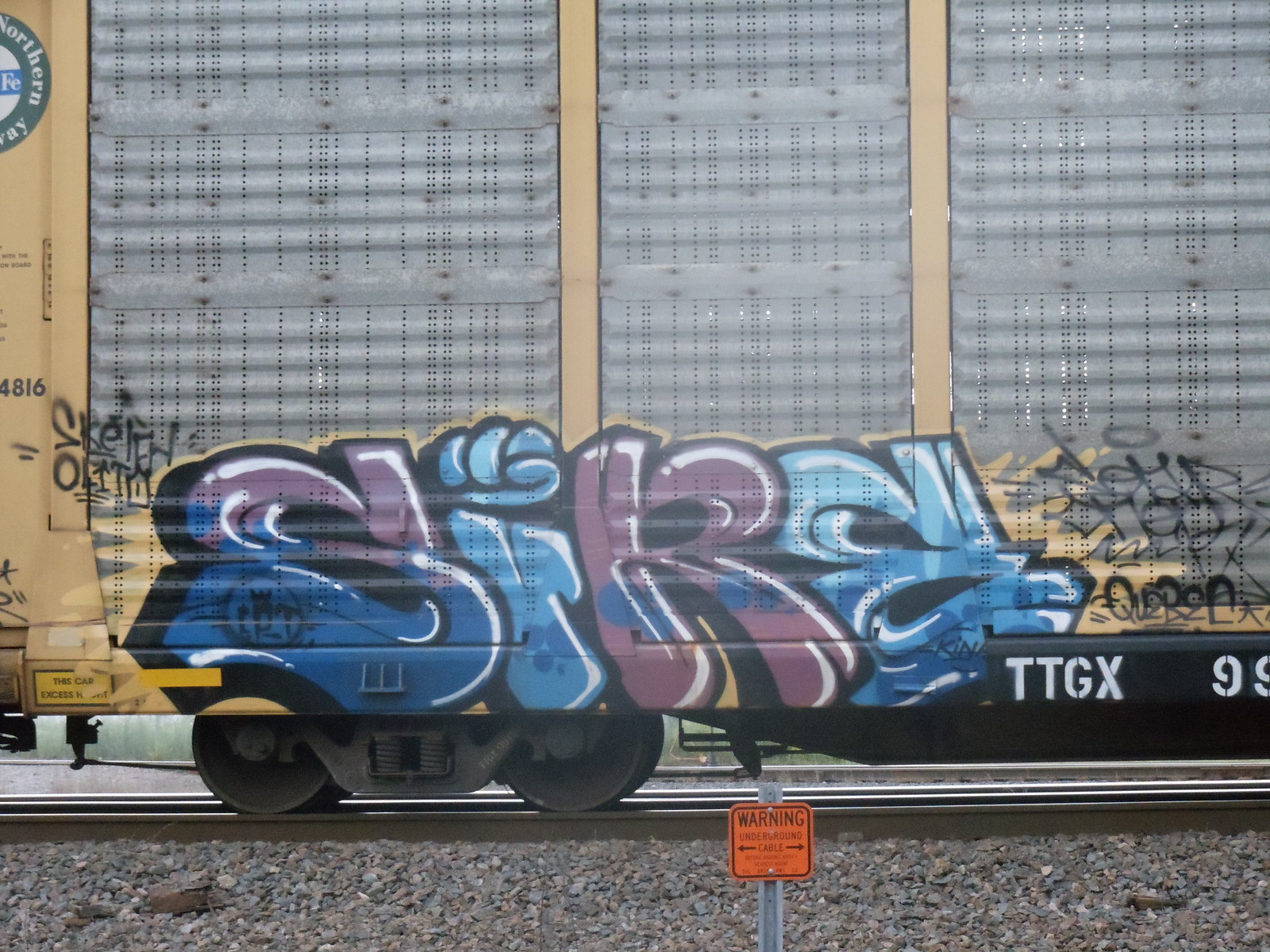The image depicts a well-maintained yellow train car, prominently featuring a set of large, silver, garage-like doors. Centered at the lower part of the train car is vibrant graffiti in blue and purple bubble letters spelling out "SIRE," with a unique clenched fist dotting the 'I'. Additional black graffiti is visible to the right of the primary text. Positioned towards the lower part of the image is an orange warning sign, partially legible with text likely indicating the presence of an underground cable. The train car rests on tracks surrounded by rocky terrain, enhancing the rugged setting. Notably, official markings are visible on the right-hand side, specifically "TTGX99," distinguishing it from the graffiti. The upper left corner of the train car also shows part of a circular logo with the letters "Northern" and a partial "Y".